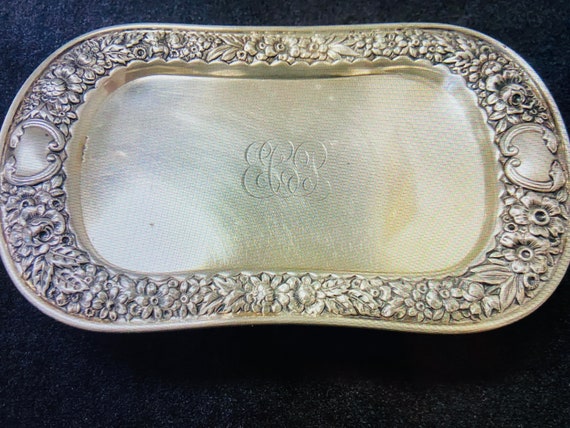A close-up photograph captures an ornate, oval-shaped silver serving tray set against a dark, possibly black, background. Elevated on what might be a table or a presentation spot, this tray's rim features intricate floral decorations that span an inch or two wide and include occasional heart shapes, all meticulously engraved into the metal. The base of the tray, curving downward like a shallow dish or plate, bears elegantly engraved letters, presumably "EJP," surrounded by fancy swirls. This tray combines artistic engravings of flowers, forming a delicate and detailed pattern. Despite the fanciful and detailed craftsmanship, the entire piece retains a cohesive silver hue, enhancing its elegance. The combination of overlapping comments reiterates the impression of a richly decorated, silver serving tray with an exquisite medley of letter engravings and flower motifs, all set on a contrasting black surface.